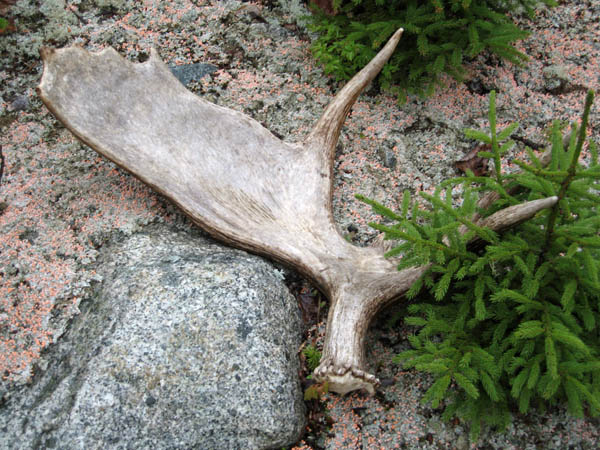This photograph captures a naturally shed moose antler lying on a pinkish-gray, sandy ground interspersed with rocks. Dominating the lower center of the image, the light tan and slightly brown antler has a large, flat portion that stretches upward and to the left, almost reaching the top left corner. It features two sharp, pointed extensions: one curving upward and to the right, and another thin point rising from the upper right side of the main stalk. To the antler's immediate left is a prominent rock, while a small, fir-like plant partially obscures the thin horn on the right. The surroundings include scattered stones, an orange-tinged sandy ground, and patches of greenery, adding to the rugged, naturalistic scene.